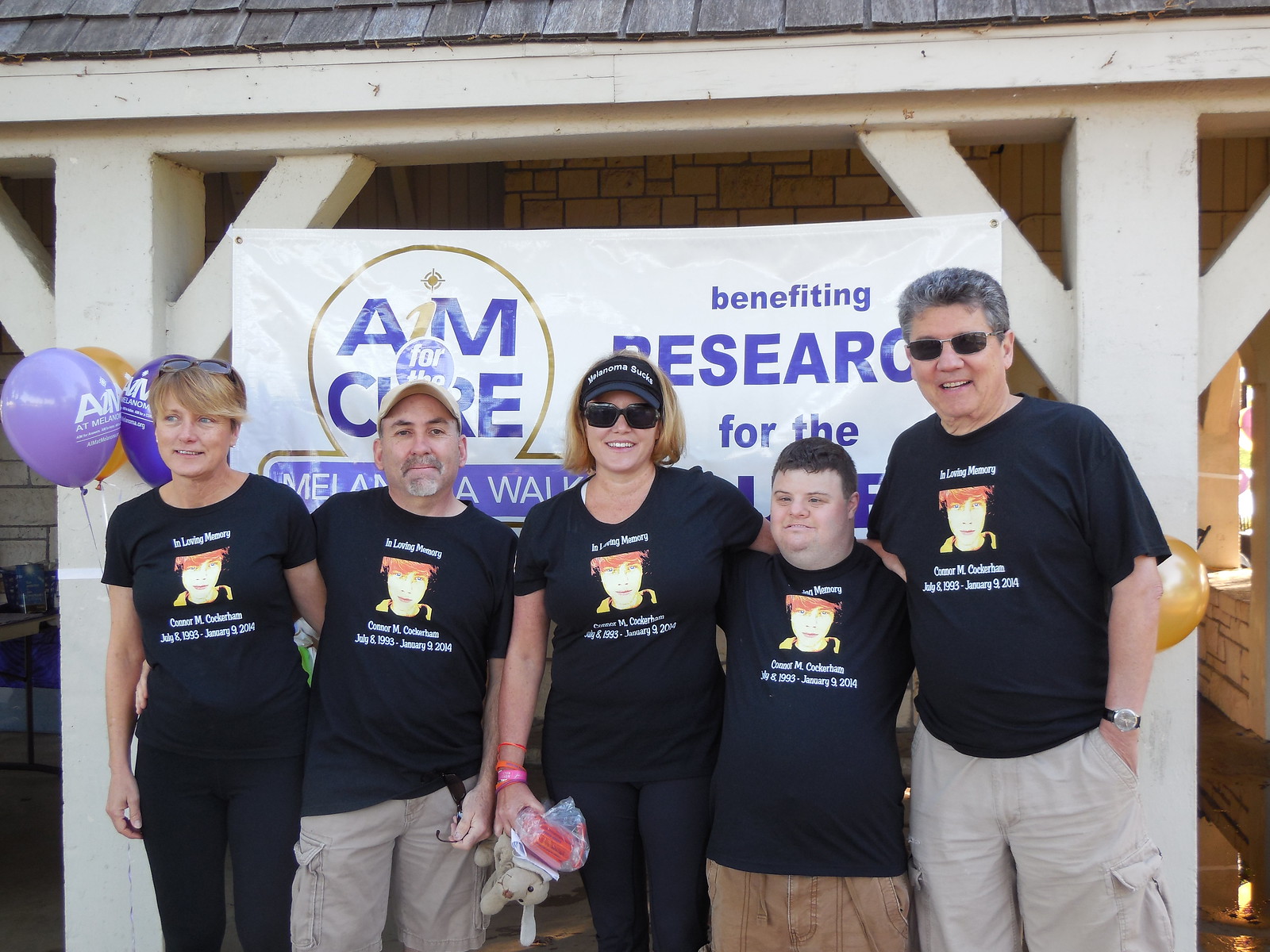In this color photograph, five people stand side by side, smiling and looking at the camera. The image features a woman, a man, a woman, a man, and another man from left to right, all dressed in identical black t-shirts with a graphic depicting a person's face, accompanied by white text that reads "In Loving Memory" along with their birth and death dates. They appear close, with some wrapping their arms around each other. The group stands outdoors in front of a building, possibly a park shelter, adorned with colorful decorations including purple and gold balloons. Behind them, a white banner, partially obscured by the group, displays a circular logo with the words "AIM FOR CARE" and additional text suggesting "BENEFITING RESEARCH." One of the women, wearing a black visor, holds a teddy bear and a package, enhancing the commemorative atmosphere. The scene suggests a fundraiser or charity event in memory of a person named Caesar who passed away on January 9, 2014, potentially to raise awareness and funds for melanoma research.